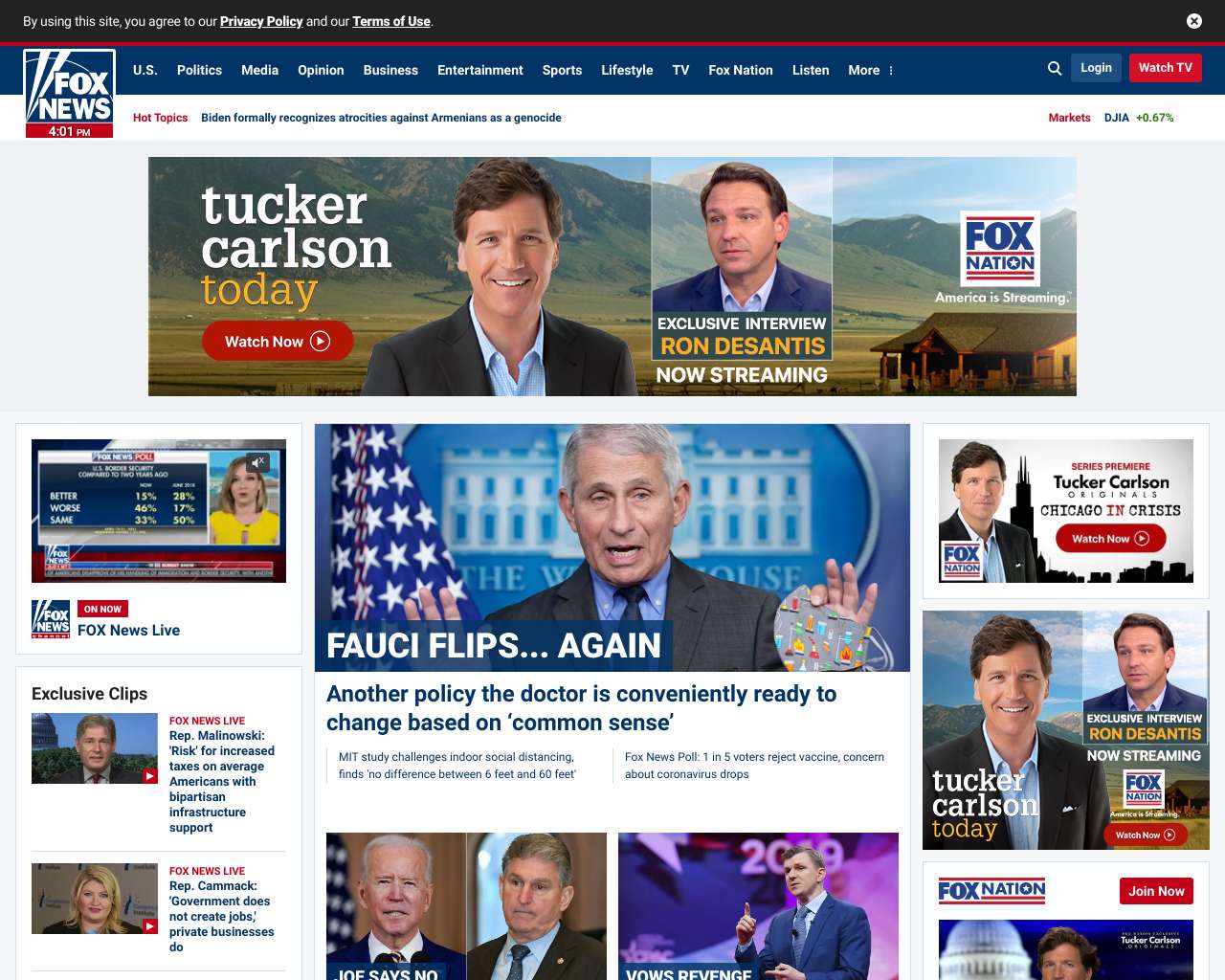This vertical image is a screenshot of a Fox News web page, which appears to be accessible on both computers and smart devices. 

At the top of the page, there's a long, narrow black rectangle with white text stating, "By using this site, you agree to our Privacy Policy and our Terms of Use." Both "Privacy Policy" and "Terms of Use" are underlined and bolded. In the upper right-hand corner of this bar, there is a white circle containing a black 'X.'

A long red line separates this section from the main header. In the upper left, a blue rectangular box displays the Fox News logo. Next to it, the time "4:01 PM" is shown. Below the logo is a navigation menu with clickable options: U.S., Politics, Media, Opinion, Business, Entertainment, Sports, Lifestyle, TV, Fox Nation, Listen, and More. There is also a magnifying glass icon for search, a login button, and a red "Watch TV" button.

Highlighted in red are the words "Hot topics," followed by the headline in blue, "Biden formally recognizes atrocities against Americans as genocide."

A prominent image of Tucker Carlson against a mountainous backdrop is featured, with the text stating, "You can watch now: Tucker Carlson Today has an exclusive interview with Rob Santas. It's now streaming." Exclusive clips are displayed on the left-hand side with various people speaking.

In the middle of the page is an article headlined "Fauci flips again," while additional articles are shown at the bottom.

On the right-hand side, there are more options to watch Tucker Carlson's segments, enhancing the webpage's focus on his show.